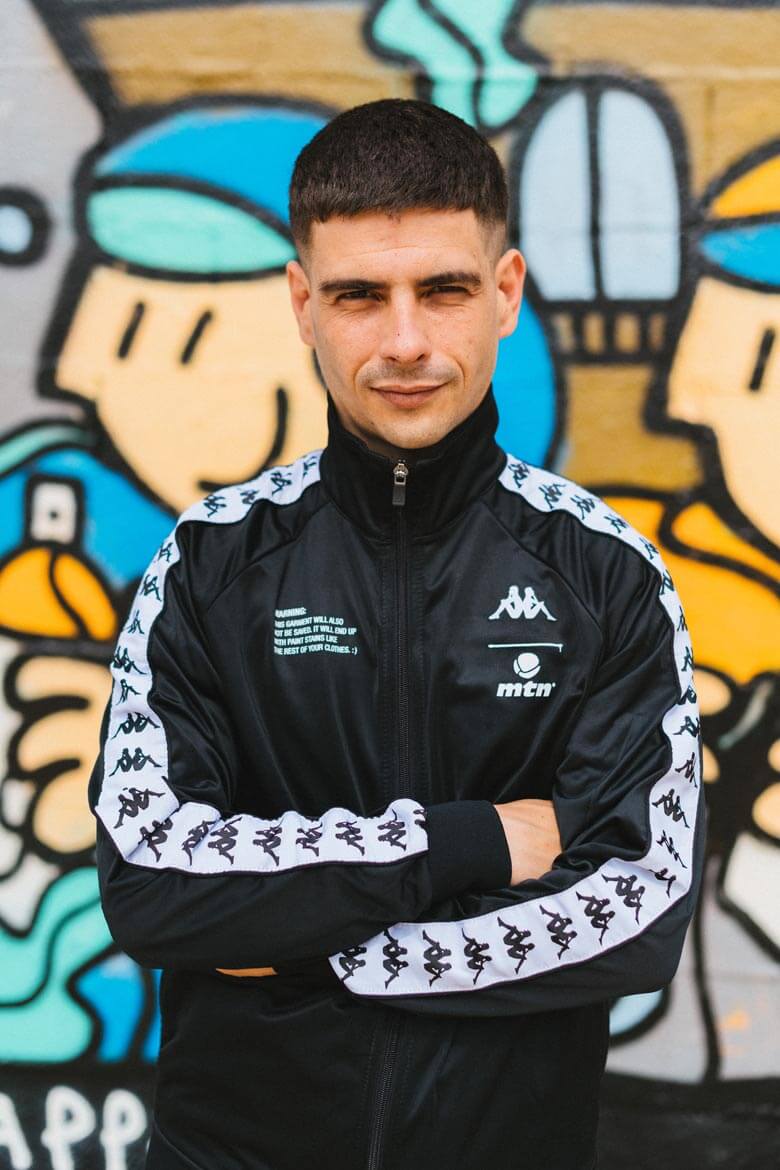The photograph captures a man, visible from the waist up, posing with his arms crossed in front of a graffiti-covered wall. The background features a vibrant mural with cartoon characters in various colors, including blue and yellow. The man, who has short black hair, narrow eyes, and a clean-shaven face, appears to be somewhat smiling as he looks directly into the camera. He is dressed in a black track jacket with a high collar and a closed silver zipper. The jacket's sleeves and chest are adorned with white lines, bearing an outline of two women sitting back to back in a repeating pattern. Additionally, on the chest, there is a white logo that reads "MTM" and white text stating, "WARNING. This garment will also not be saved. It will end up with paint stains like the rest of your clothes." The overall brightness of the image suggests it was taken on a sunny day, even though the background appears slightly blurred.